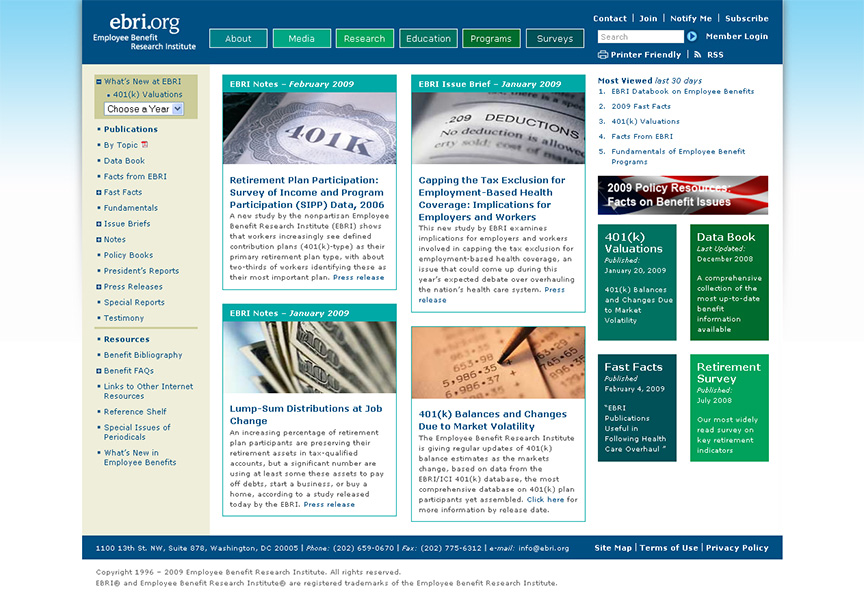**Detailed Caption for Screenshot of Employee Benefit Research Institute Website:**

The screenshot captures the homepage of the Employee Benefit Research Institute (EBRI) website, identifiable by the logo "ebri.org" prominently displayed in the top left corner. The top of the screen features a distinct blue banner adorned with various navigation elements. Central to this banner are green buttons labeled: About, Media, Research, Education, Programs, and Surveys. On the right-hand side of the banner, white text hotlinks offer quick access to: Contact, Join, Notify Me, Subscribe, Member Login, Printer Friendly, and RSS, alongside a search box for user convenience.

To the left of the main content, there is a vertical menu in a beige or yellowish hue, which begins with a section titled "What's New at eBRI." Below this are options such as "401k Valuations" and a dropdown box labeled "Choose a Year." Further down the menu, more detailed navigation options include: Publications, My Topic, Data Book, Facts from eBRI, Fast Facts, Fundamentals, Issue Briefs, Notes, Policy Books, President's Reports, Press Releases, Special Reports, Testimony, Resources, Benefit Bibliography, Benefit FAQs, Links to Other Internet Resources, Reference Shelf, Special Issues of Periodicals, and What's New in Employee Benefits.

At the bottom of the screen, another blue banner provides essential contact information including the address, phone number, fax number, email address, and links to the site map, terms of use, and privacy policy. The footer also contains copyright information.

Dominating the center of the screen are four featured articles, split into two rows. The top row highlights "eBRI Notes, February 2009" with a focus on "Retirement Plan Participation, Survey of Income and Program Participation (SIPP) Data 2006," and "eBRI Issue Brief, January 2009" detailing "Capping the Tax Exclusion for Employment-Based Health Coverage: Implications for Employers and Workers," both accompanied by explanatory descriptions and generic stock photos of financial documents and instruments. 

The bottom row includes "eBRI Notes, January 2009" about "Lump Sum Distributions at Job Change" and another article titled "401k Balances and Changes Due to Market Volatility," each accompanied by concise descriptions and relevant stock imagery.

To the right, there is a sidebar featuring two key sections: a box listing the most viewed articles in the past 30 days, and a box displaying an American flag with a label for "2009 Policy Resources." Below this, four additional boxes provide links to specific resources: 401k Valuations, the Data Book, Fast Facts, and a Retirement Survey.